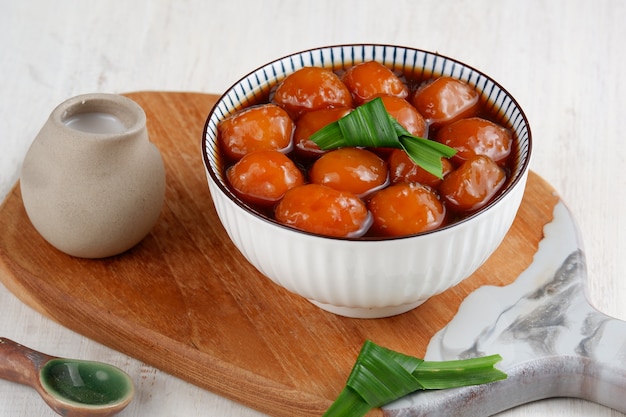In the bottom left corner of the image, there is a wooden spoon with a green-tinted interior, positioned next to a small white jar that may be empty. Both items rest on a wooden and marble display board. Dominating the center of the image is a pristine white bowl, artfully presented. Inside the bowl is a fresh green leaf serving as a base for the vibrant orange, circular objects. This colorful and artistic arrangement showcases a traditional Indonesian dessert porridge, known for its sweet and unique flavors. The scene is meticulously organized to highlight the exotic and visually appealing elements of the dish.